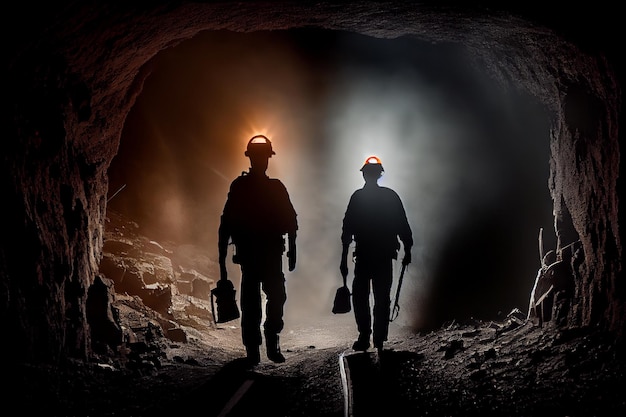In this photo, two men, possibly coal miners, are captured walking deeper into a dark cave. They are wearing hard hats equipped with lights—one emitting an orange glow and the other a light blue. Their silhouettes reveal that they are in full work attire, including boots, long pants, and long-sleeve shirts. One man appears to be carrying a long object, potentially a shovel, while both seem to have small backpacks. The cave's rough, rocky walls and uneven ground surround them, with the darkness enveloping the scene and their lights illuminating the path ahead. The contrast between the pitch-black environment and the glowing headlamps highlights the rugged, enigmatic nature of their surroundings.